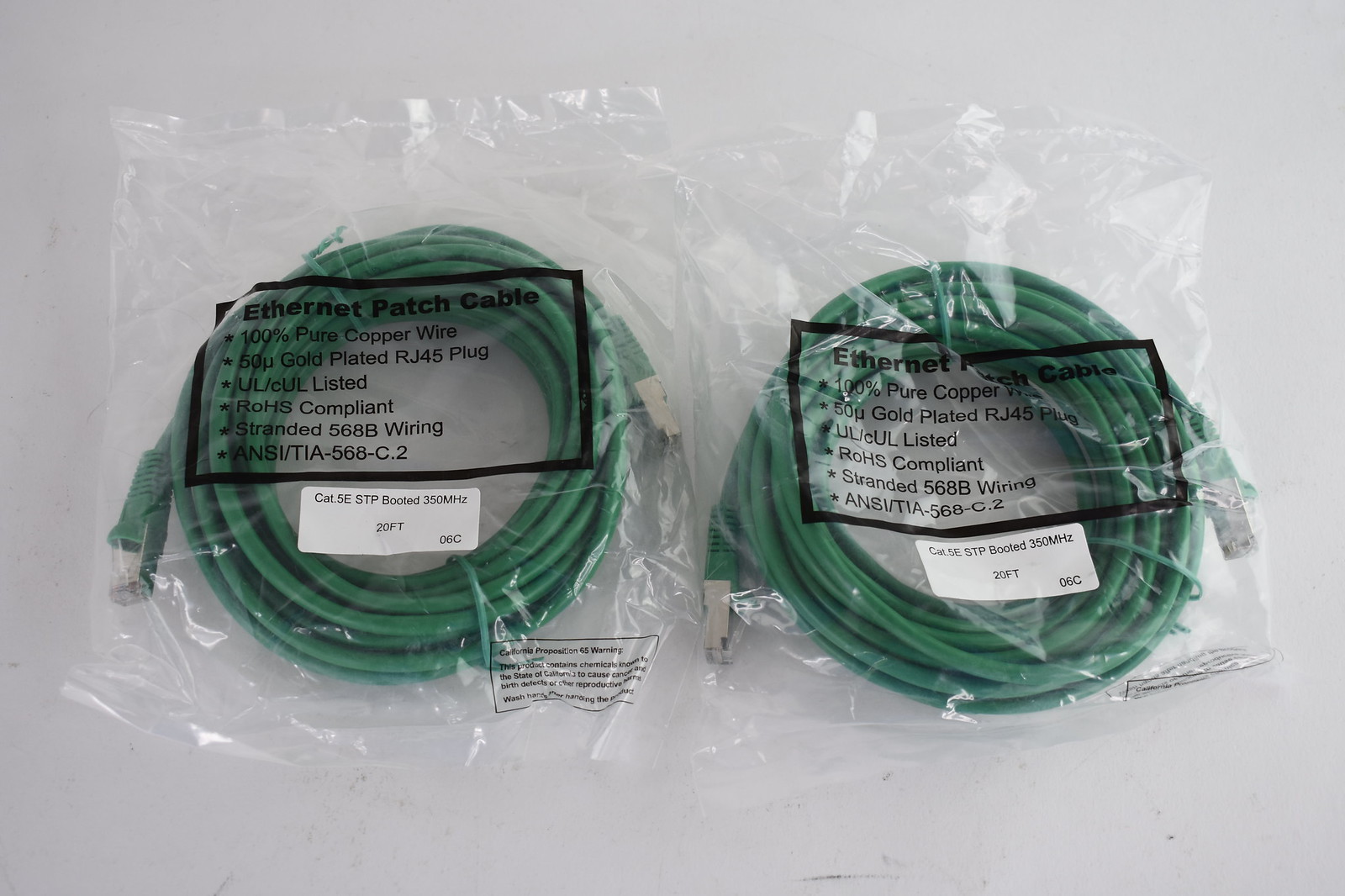On a white background, we see two vacuum-sealed plastic pouches containing green Ethernet patch cables, meticulously looped and secured with wire ties. Each package prominently features detailed specifications printed in black ink: the cables are constructed from 100% pure copper wire and equipped with gold-plated RJ45 plugs, UL/CUL listed, and ROHS compliant. They adhere to ANSI/TIA-568-C.2 standards with stranded 568B wiring. Additional details on a white sticker indicate that these are Cat5e cables, SEP booted, supporting up to 350 MHz frequencies, and measure 20 feet in length.